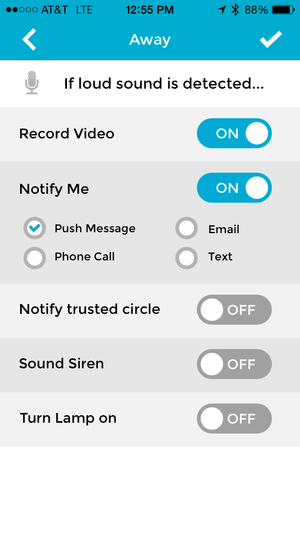This is a screenshot of a cell phone display taken at 12:55 PM, as indicated by the time at the center of the top bar. The status bar is a gradient transitioning from blue to light blue to an aqua color. The device shows two out of five dots for cell signal strength, indicating reception. It is an AT&T phone connected to an LTE network, with the battery level at 88%. A Bluetooth icon is also visible in the status bar.

The current page displayed on the phone is titled "Away," set against a white background. The interface indicates, "If loud sound is detected," accompanied by a gray microphone icon to the left of the text. Below this, the screen shows several settings with their respective toggles: 
- "Record Video" is activated.
- "Notify Me" is also activated, with an additional option, "Push Message," checked.
- "Notify Trust Circle" is deactivated.
- "Sound Alarm" is deactivated.
- "Turn Lamp On" is deactivated.

The detailed display suggests a security or monitoring application in use, with multiple notification and response settings configured.